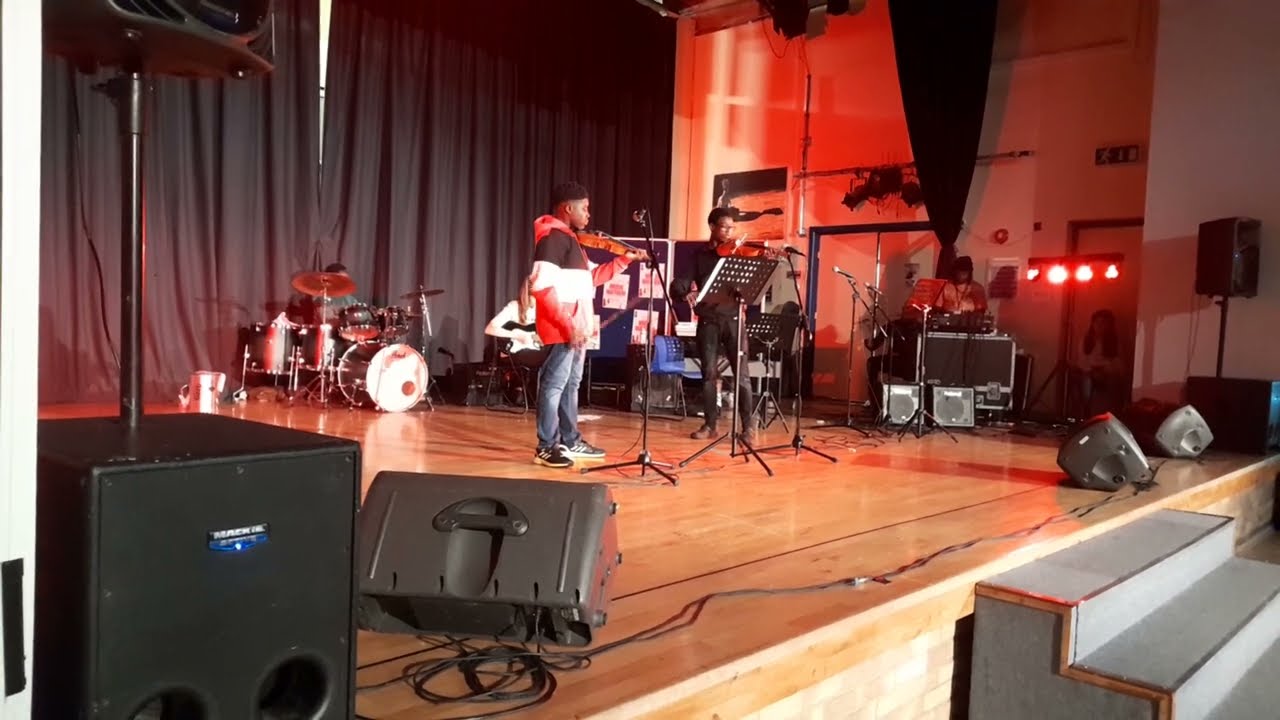The image captures a vibrant stage scene with a wooden floor, partially visible through the red-tinted light flooding the setting. From the bottom right corner, portable gray steps lead up to the stage. Dominating the left side of the image are large speakers placed at an angle that diminishes towards the center right. 

Central to the scene are two young men playing violins. The man on the left, a young Black male with dark hair, dressed in a black, white, and red jacket, blue jeans, and black sneakers, passionately plays his violin in front of a microphone on a stand. To his right, another man, casually attired in blue jeans, black Adidas sneakers, and a large hoodie with a red hood, holds his violin and bow but is not actively playing. 

Further to the right, partially obscured by equipment, a person wearing a cap sits behind what appears to be a computer, potentially managing the stage's technical aspects. 

The backdrop features tall black curtains and to the left behind the violinists, a drummer is seated at a drum set. The stage is framed by an arrangement of bright red lights, especially noticeable near the exit doors on the right, casting a warm glow over the entire scene.